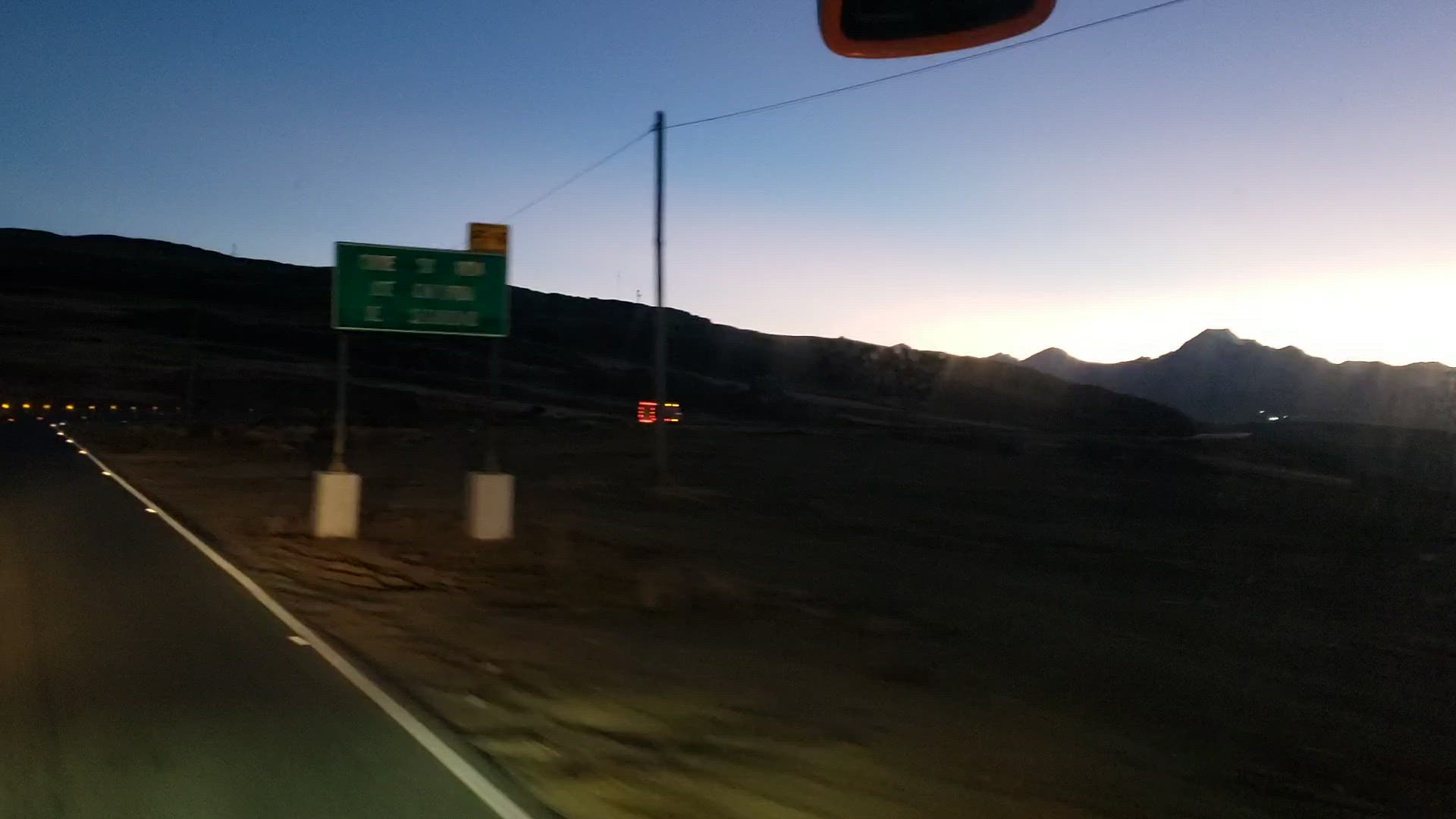This photograph, likely taken from a moving vehicle, captures a desolate stretch of road that extends into a vast desert landscape. The black asphalt of the road contrasts starkly with its lightly gravelled shoulder. There are no other vehicles in sight, emphasizing the solitude of the scene. To the right side of the road, a green street sign, blurry and indistinct, hints at upcoming destinations with white lettering. Adjacent to the sign, power lines trail off into the distance, adding to the sense of remoteness. The backdrop features a barren desert devoid of trees or buildings, stretching out to the distant outline of mountains. The sky is tinged with the warm hues of dusk, reflecting the approaching night as the sun sinks below the horizon.